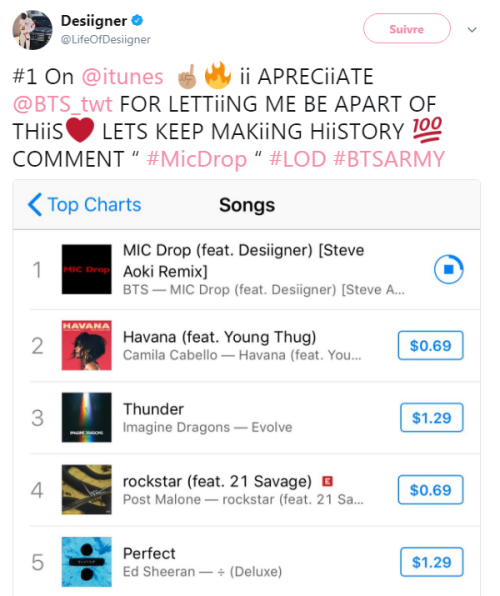**Caption for the Image:**

This is a detailed screenshot from a social media profile and music chart listing. At the top, there is a user profile featuring a round photo and the name "DESIIGNER" in bold, accompanied by a blue verified checkmark. The handle "@lifeofdesigner" is displayed prominently, with a “SUIVRE” button (French for "Follow") accompanied by a dropdown arrow to the right.

The post by DESIIGNER enthusiastically announces that their track is "number one on @iTunes," highlighted with a number one finger and flaming emojis. The text uniquely uses double I's, likely a branding choice by the designer. The message reads: "II appreciate @BTS_TWT for letting me be a part of this. II love you! Let's keep making history!" followed by a heart emoji and a 100 emoji. The post concludes with hashtags: #micdrop, #LOD, and #BTSARMY, indicating strong affiliation with the BTS fan community.

The screenshot includes a menu titled "Songs," showcasing the "Top Charts" section highlighted in blue with a left arrow. Five songs are listed, each with a square profile image. At the top is "MIC Drop (Steve Aoki Remix)" by BTS featuring DESIIGNER, and it has a play button next to it. The following songs are:
1. "Havana" by Camila Cabello featuring Young Thug – $0.69
2. "Thunder" by Imagine Dragons – $1.29
3. "Rockstar" by Post Malone featuring 21 Savage – $0.69
4. "Perfect" by Ed Sheeran – $1.29